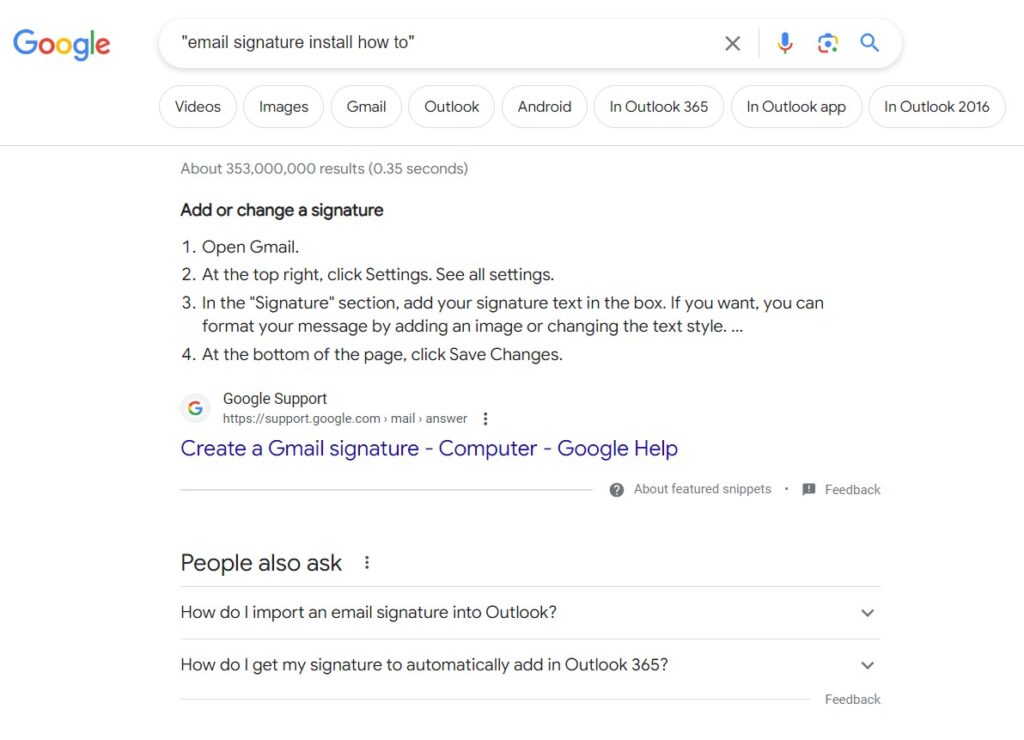The image showcases Google search results for the query "email signature install how-to." Positioned at the upper left is the recognizable Google logo. Within the search field, the query is enclosed in quotes, and to the right are icons: an 'X' to clear the search, a microphone for voice search, a camera for image search, and a magnifying glass to initiate the search.

Below the search bar, there's a tabbed menu that includes options like 'All,' 'Videos,' 'Images,' 'News,' and 'More.' Highlighted are distinct results for Gmail, Outlook, Android, Outlook 365, and Outlook app in Outlook 2016. The search yields approximately 353 million results in 0.35 seconds.

The first result is prominently displayed with a bold title: "Add or Change a Signature." It outlines four clear steps:
1. Open Gmail.
2. At the top right, click Settings and then See all settings.
3. In the Signature section, add your signature text in the box, with options to format your message by adding an image or changing the text style.
4. At the bottom of the page, click Save Changes.

This information is sourced from Google Support, evident from the link title "Gmail signature - computer - Google Help." Additionally, the "People also ask" section features two questions: "How do I import an email signature into Outlook?" and "How do I get my signature to automatically add in Outlook 365?" The rest of the screen remains white, adhering to Google's minimalist design aesthetic.